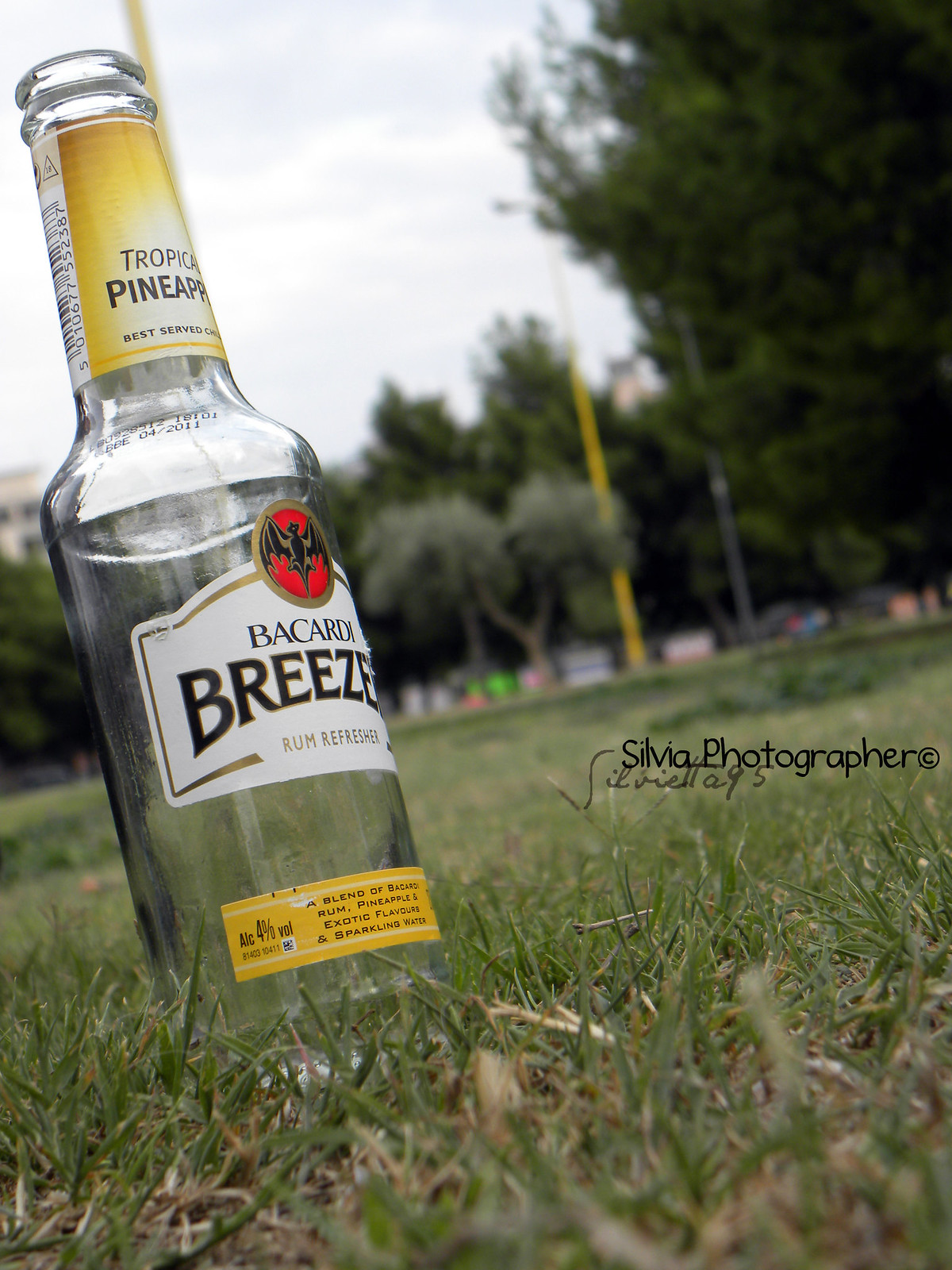This detailed professional photograph by Sylvia Photographer captures a Bacardi Breeze Rum Refresher Tropical Pineapple bottle resting on grassy ground. The bottle, positioned on the lower left side of the frame, tilts slightly to the left and features a distinctive design with a yellow and white label on the neck and a prominent white label emblazoned with the Bacardi logo—a red circle emblem—on the main body. Additionally, the bottom part of the bottle sports a yellow label detailing the contents. The image emphasizes a close-up perspective, showcasing individual blades of grass around the bottle. The backdrop features a blurry setting of a park, with hints of green trees and indistinct playground elements. On the right side of the image is a visible copyright notice, "Sylvia Photographer ©".